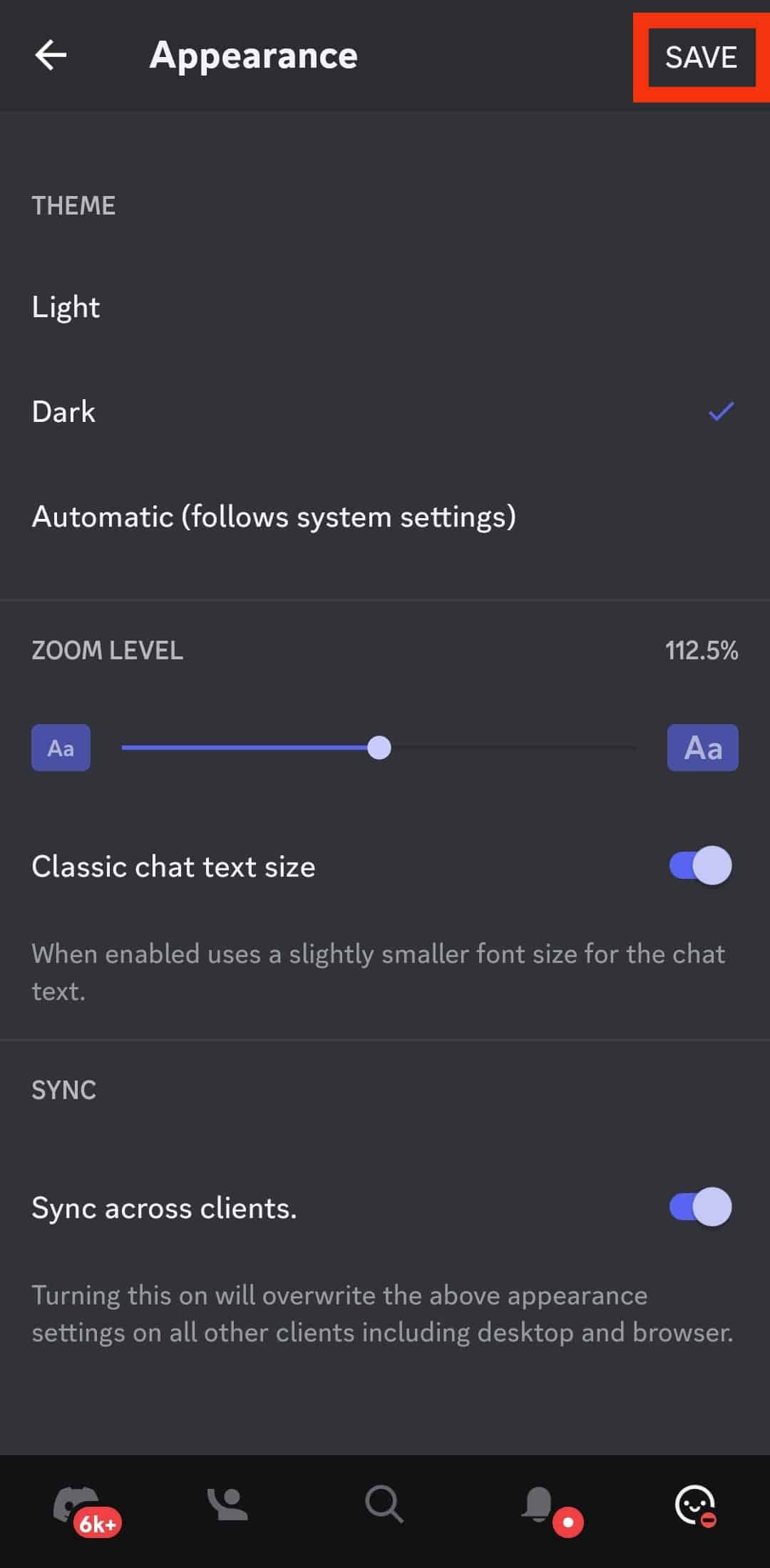This is a screenshot from an Android device's settings menu, displaying the "Appearance" category in dark mode. The background is nearly black with white text at the top reading "Appearance." Below that, the section labeled "Theme" presents options to select either "Light" or "Dark" mode, with a blue checkmark indicating that "Dark" mode is currently active. The next section shows the "Zoom level," set at 112.5% with an adjustable slider. The slider is positioned halfway, illustrated by a half-blue, half-clear bar. Further down, there's an option for "Classic chat text size," which features a blue toggle switch in the "on" position. Finally, the "Sync across clients" option, also with a blue toggle switch turned on, is displayed at the bottom of the screenshot.